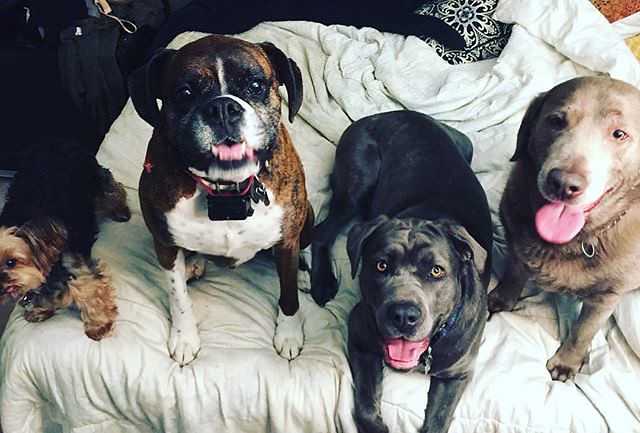In this rectangular image, four distinct dogs are comfortably arranged on a bed covered with a white, tousled sheet that drapes over the edge. At the back of the bed, a separate piece of black material spans from the top left corner to about three-quarters of the way to the right. On the far left side of the image, partly cut off, stands a small Yorkshire Terrier with gray and black fur, gazing off into the distance. To the right of the Yorkie is a brown Bulldog with a white chest and paws, featuring some black around its eyes and ears, and its mouth slightly open. Next to the Bulldog, lying down with legs hanging over the bed’s edge, is a black dog resembling a Black Labrador, its mouth open and pink tongue visible. The far right displays an older light tan dog with a very brown nose, enthusiastically panting with its tongue protruding. All four dogs appear to be of different breeds, facing the camera, and wearing collars, adding a layer of charm to this cozy, canine ensemble.